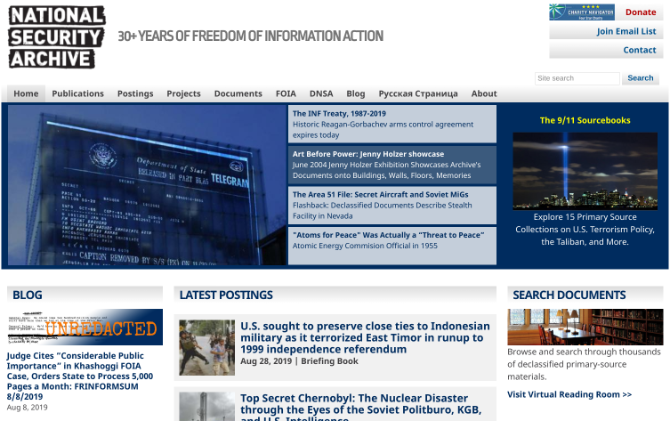The screenshot depicts the homepage of the National Security Archive’s website, conveying a structured layout designed to provide extensive information on various topics. 

In the upper left corner, the header features the title "National Security Archive" in white font over a series of three dark rows. To the right of the title, it states "30+ Years of Freedom of Information Action." Adjacent to this text is a red "Donate" button and below it, a "Join Email List" button followed by a "Contact" link. Beneath these buttons, there is a site search input field accompanied by a blue search button.

Directly below the National Security Archive header, there is a navigation menu with multiple tabs, including "Home," "Publications," "Postings," "Projects," "Documents," "FOIA," "DNSA," "Blog," and an additional tab with Cyrillic text, likely representing Russian content, followed by an "About" tab. The "Home" tab appears to be selected, indicated by a highlighted background.

The main content area features a series of articles. On the left side, there is a thumbnail image, including an electronic writing or a 3D image of a building with a video wall displaying the word "Telegram." The articles span various historical and topical subjects:

1. "The INF Treaty From 1987 to 2019" - Highlights the expiration of the historic Reagan-Gorbachev arms control agreement.
2. "Art Before Power: Jenny Holzer Showcase, June 2004" - Focuses on Jenny Holzer’s exhibition that showcased archival documents projected onto buildings, walls, floors, and memories. This article stands out with a light navy background, indicating it is currently selected.
3. "The Area 51 File: Secret Aircraft and Soviet MiGs" - Discusses declassified documents describing the stealth facility in Nevada.
4. "Atoms for Peace Was Actually a Threat to Peace" - Features commentary from an Atomic Energy Commission official in 1955.
5. "The 9-11 Terrorist Books" - Explores 15 primary source collections on U.S. terrorism policy and the Taliban, accompanied by an image of the New York skyline at night, with a blue beam rising from the ground, symbolizing the Twin Towers’ original location.

The detailed structure and layout underscore the National Security Archive’s commitment to transparency and education through its comprehensive repository of documents and exhibitions.